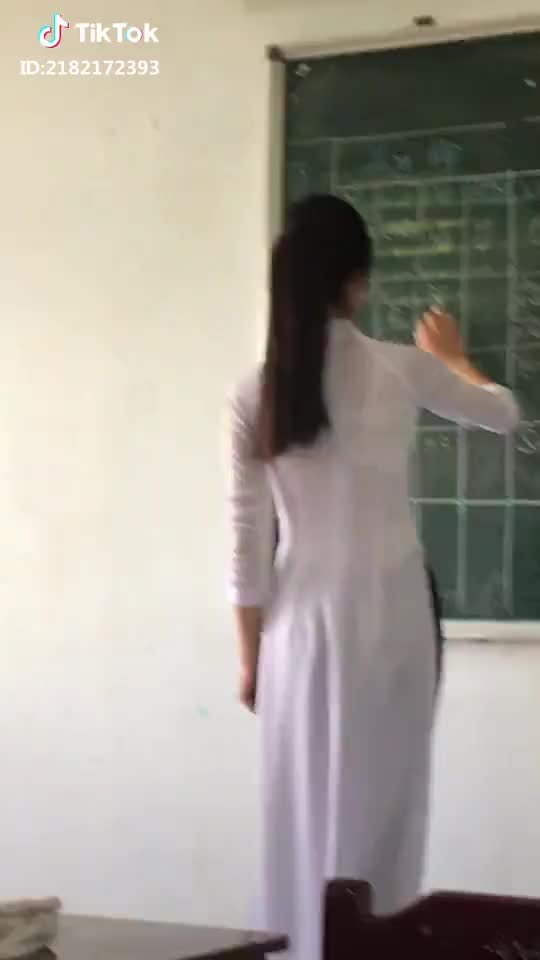The image depicts a vertical, rectangular scene of a teacher writing on a green chalkboard, which is framed by a silver metal border. The chalkboard starts from the center of the background to the right. The teacher, with her back turned to the camera, is writing with a white piece of chalk. Due to the blurriness, the specific content she is writing, which appears to include a table or grid lines, is indiscernible. She has dark black, straight hair tied in a ponytail that reaches the middle of her back. She is dressed in a long, white outfit with sleeves that extend to her elbows and a neckline that sits high. The tops of brown wooden desks and chairs are visible at the bottom edge of the image. In the upper left-hand corner, there is a white TikTok logo, below which is the text "ID: 218-217-2393". The image quality is low and seems to be a screenshot from a video.